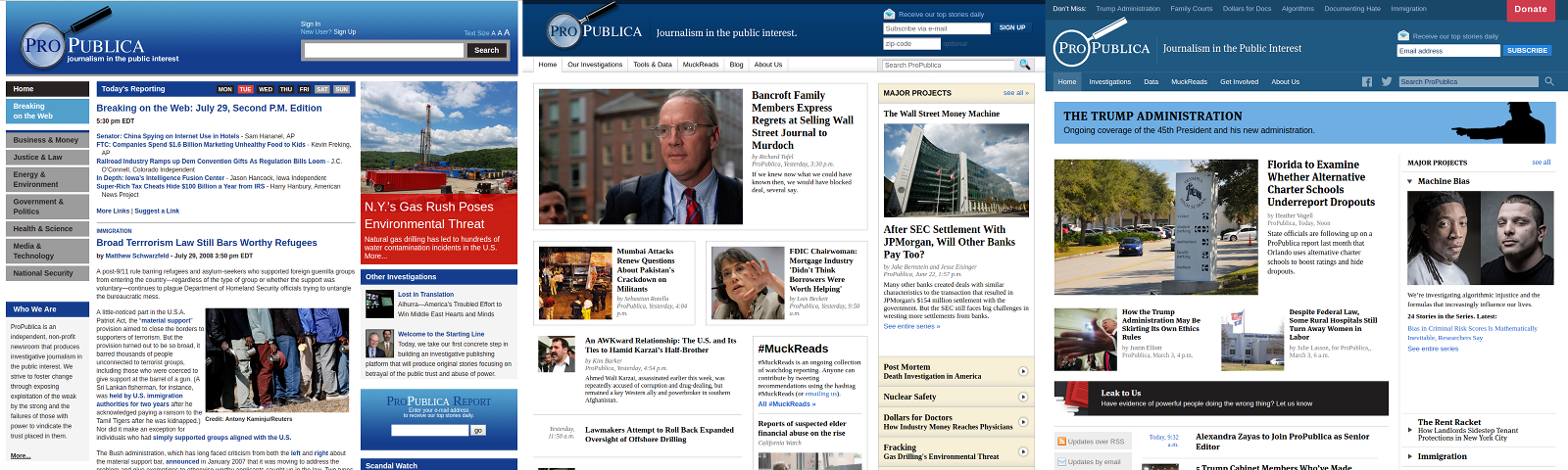This photo is a collage featuring three front pages of the ProPublica website, showcasing its evolution over time. Each page is squared and arranged horizontally side by side, forming a large rectangular composite.

- **First Page (Leftmost)**
  - **Header**: Light blue with the ProPublica logo on the left.
  - **Left Panel**: Categories listed.
  - **Main Content**: Two central articles (one top, one bottom).
  - **Right Side**: A large advertisement in the top right with additional articles below it.

- **Second Page (Middle)**
  - **Header**: Thinner and darker blue with the ProPublica logo in the top left and a sign-in box to the right.
  - **Left Side**: Thumbnails accompanying article links.
  - **Right Side**: Categories with drop-down boxes for minimization, revealing articles within each category.

- **Third Page (Rightmost)**
  - **Header**: Thicker and a darker blue.
  - **Below Header**: A large light blue banner featuring a compilation of archived stories.
  - **Content**: Thumbnails and articles displayed on both the left and right sides of the page.

This collage visually captures the design and layout changes of the ProPublica website over different periods.